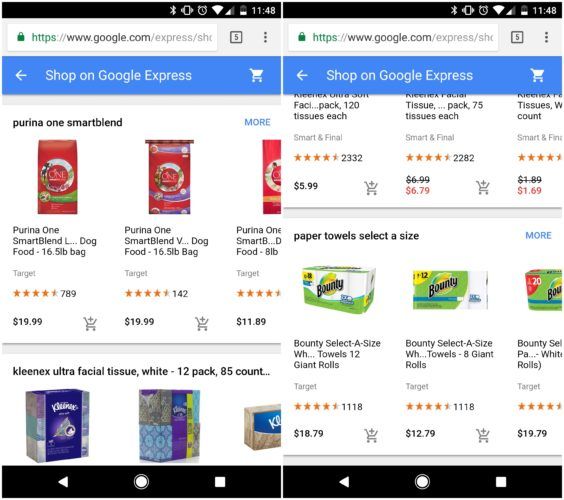The image showcases Google Express search results displayed on two different phone screens, captured in separate screenshots. The screenshot on the left features a search for Purina One SmartBlend products. The results are presented in a tabulated format with the following options:

1. Purina One SmartBlend (16.5 pounds) priced at $19.99.
2. Purina One SmartBlend (16.5 pounds) also priced at $19.99.
3. Purina One SmartBlend (8 pounds) priced at $11.85.

Below these listings, a product entry for Kleenex Ultra Facial Tissue is visible, specifically a white 12-pack with 85 counts per box. Three different images of this Kleenex product variety are included.

The right-side screenshot appears to continue from the left, showing further results as if the original screenshot was scrolled down. It includes a variety of Bounty Towels:

1. Bounty Towels (12 Giant Rolls) priced at $18.79.
2. Bounty Towels (8 Giant Rolls) priced at $12.79.
3. Another variant of Bounty Towels, although the description is partially cut off, priced at $19.79.

Both screenshots indicate that these products are offered through Google Express with Target serving as the retailer, as denoted by the Target label in each product cell. Each product listing also includes user rating averages represented by orange stars, with the number of reviews ranging from hundreds to thousands.

The overall background of both screenshots is white, providing a clean and uncluttered browsing experience.